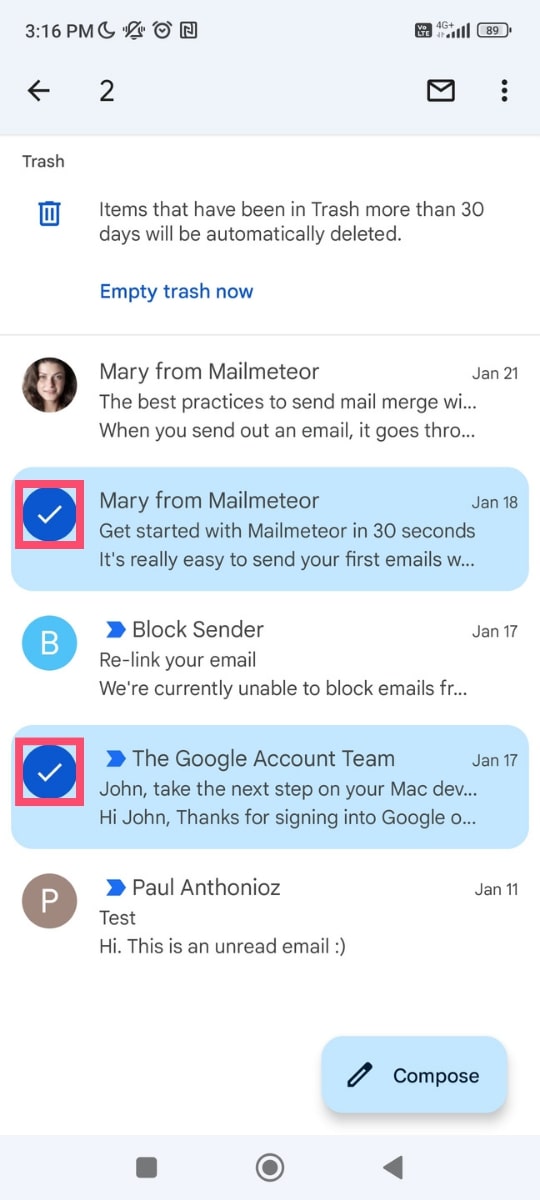The image depicts a Gmail inbox interface with a notification banner at the top stating, "Items that have been in Trash more than 30 days will be automatically deleted. Empty trash now." Below the banner, several emails are visible:

1. An email from "Mary at MailMeter" with the subject: "The best practice is to send Mail Merge, and when you send an email it goes through."
2. Another email from the same sender, "Mary at MailMeter," with the subject: "Get started with Mail Meter in 30 seconds; it’s really easy using your first emails."
3. An email with the subject line indicating a warning: "Block sender: Relink your email. We're currently unable to block emails."
4. A communication from the "Google Account Team" with the subject: "John, take the next step on your Mac. Hi John, thanks for signing into Google."
5. The final email is from "Paul Antonio," with the subject: "Hi, this is an Irony mail."

This detailed caption provides a comprehensive view of the contents and context of the image.